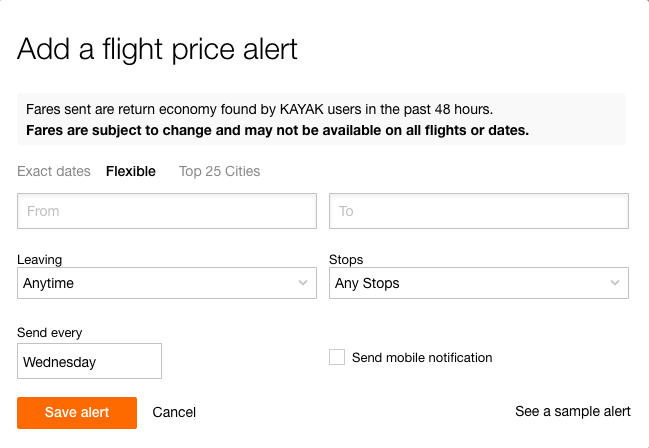The image is a screenshot of a web page with a white background and black text. At the top, in prominent black letters, it reads "Add a flight price alert." Below this header, a smaller text indicates, "Fares sent are return economy found by Kayak users in the past 48 hours. Fares are subject to change and may not be available on all flights or dates."

A user has interacted with this page, selecting "Flexible" as their preference. Further down, the page features two input boxes labeled "From" and "To," which indicate the departure and destination locations.

Below these fields, there's a section titled "Leaving," with a box beneath it in which the user has entered "Any time." Next, there's a "Stops" section, where the user has selected "Any stops" in a corresponding black box.

Toward the bottom left of the page, there's a prompt that says "Send every," followed by a text box where the user has entered "Wednesday." This indicates that the user wishes to receive price alerts on flights every Wednesday. 

Finally, in the bottom right corner of the image, there's a large orange rectangle button with the words "Save alert" written on it in white text. This button is likely intended for users to finalize and save their flight price alert settings. 

Overall, the user is setting up a flexible flight price alert to receive notifications for any flights, with any number of stops, departing on any date, and to be alerted about these on Wednesdays.